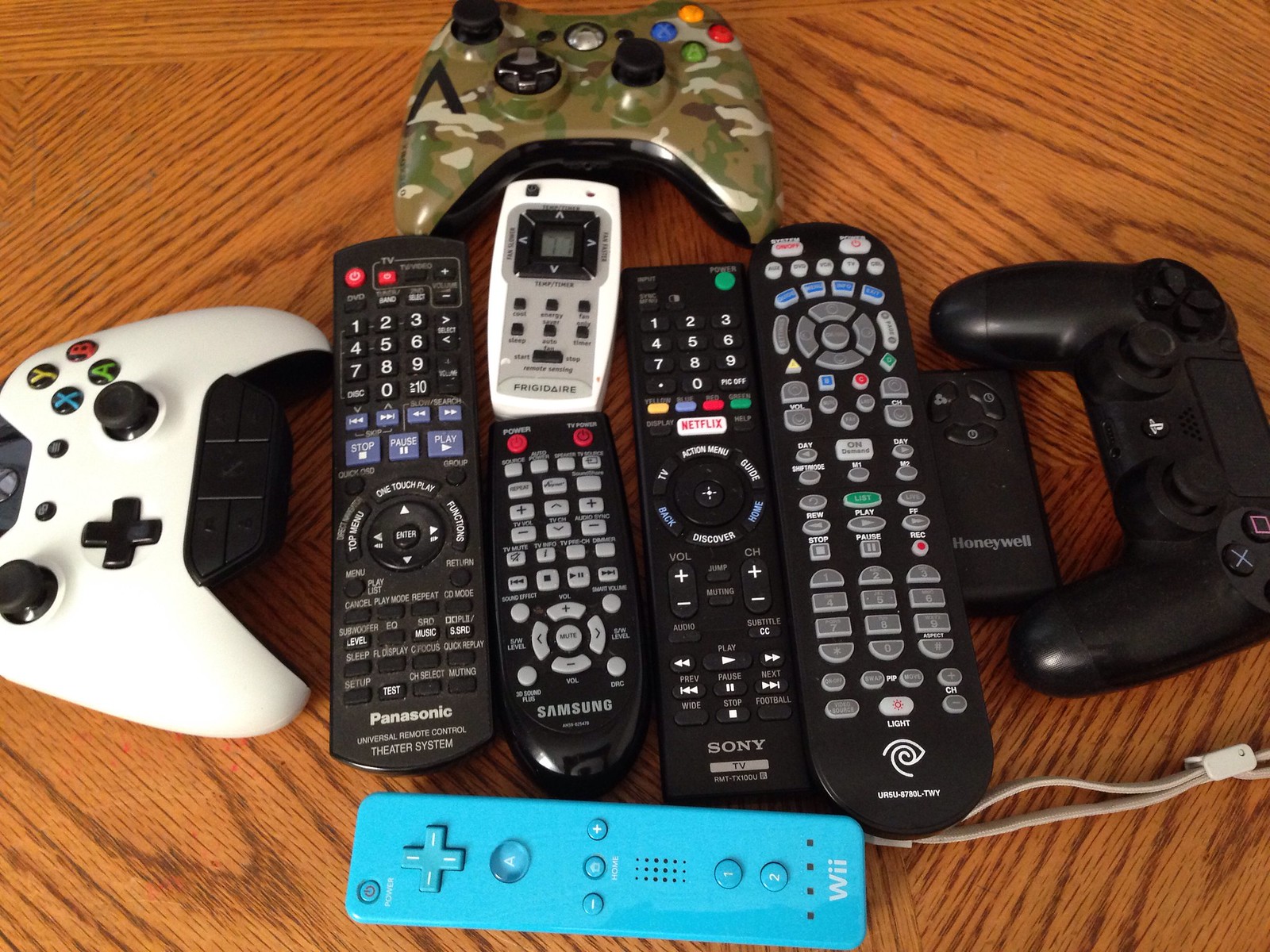In this image, the background is a light brown wooden table. Various remotes and game controllers are scattered across the table. At the forefront, there's a light blue Wii controller with "Wi-Fi" or "Wii" written at the bottom, positioned in the lower right corner. Surrounding it, at the left edge, is a white Xbox controller, and on the right edge, a black PlayStation controller. Towards the top center lies a camouflage-colored Xbox controller adorned with yellow, red, blue, and green buttons.

In the middle section, there are at least five different black remotes, including one with a Sony logo, one marked Samsung, another labeled Panasonic, and another with a swirl design. There's also a small miniature Honeywell remote. Additionally, a Frigidaire remote stands out with its white frame and gray body. Among these controllers, one has a cord attached, hinting at a wired connection. The large black remotes feature many buttons in various colors, including arrow keys and buttons labeled with services like Netflix. This eclectic collection reveals a control hub for an extensive entertainment system, laying command over multiple devices.